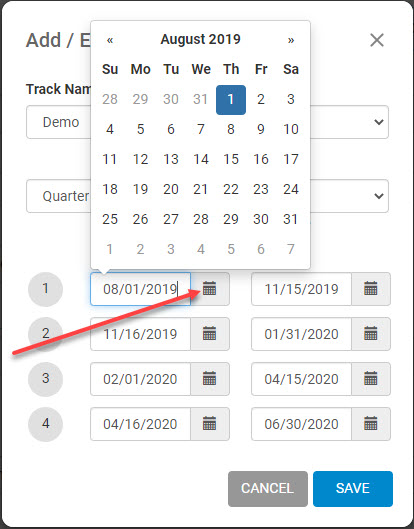This image features an emergency calendar highlighting key dates and periods. The detailed timeline begins with Thursday, August 1, 2019, marking the start of the month, which spans from Thursday and concludes on Saturday, August 31, 2019. In the background, there is a sequence of significant dates and timeframes outlined as follows: 

1. From August 1, 2019, to November 15, 2019
2. From November 16, 2019, to January 31, 2020
3. From February 1, 2020, to April 15, 2020
4. From April 16, 2020, to June 30, 2020

Each period is sequentially numbered to aid in easy reference.